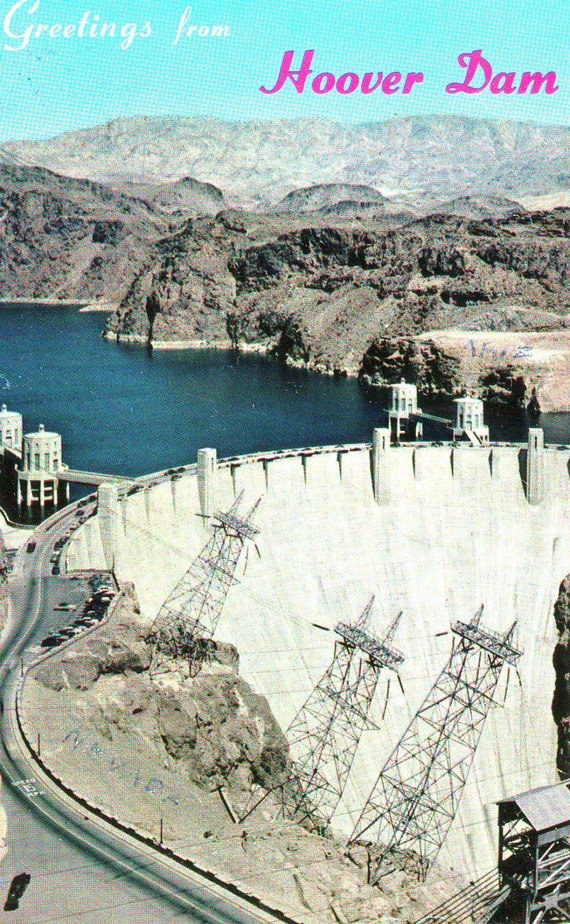This vintage postcard from the 1950s or 60s features an aerial view of the majestic Hoover Dam. The image captures the immense concrete structure of the dam, dominating the lower half of the card, with the tranquil, bluish-green water of the reservoir stretching out behind it. The dam is framed by rugged Nevada rock formations and distant mountains, under a bright blue sky. In the very foreground, we see a walkway and a road, with cars possibly parked at lookout points. Prominently positioned are several angled electrical towers and other metal infrastructures, giving a sense of the dam’s scale and engineering marvel. The top of the postcard is adorned with "Greetings from Hoover Dam," with "greetings from" in white cursive text and "Hoover Dam" in a vibrant pinkish-purple font.